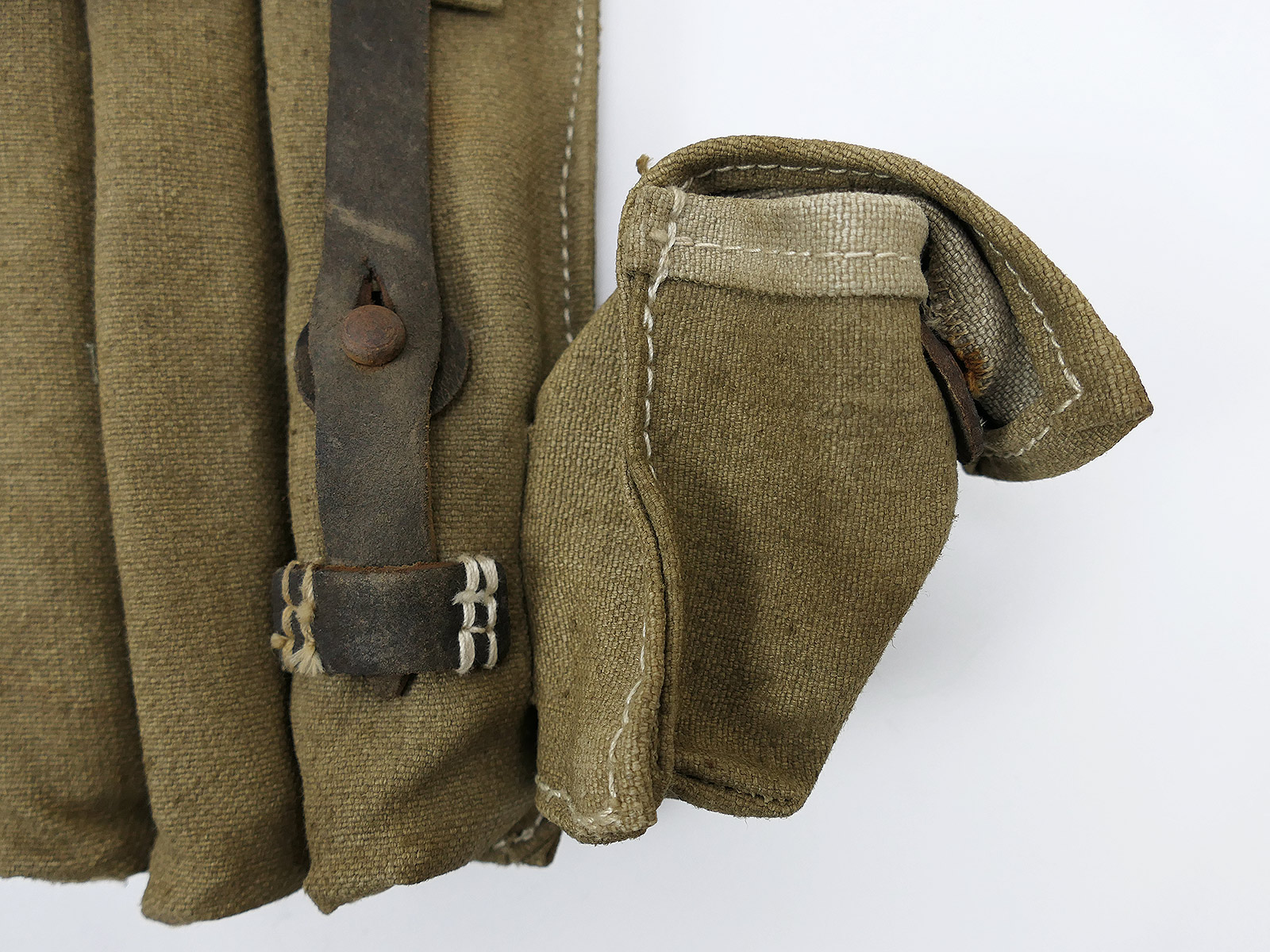The image captures a close-up of an olive green cloth item, likely a garment, set against a solid white background. The fabric, resembling either canvas or burlap, features a unique configuration of three tube-like sections sewn together in a circular shape. On the left-hand side, the cloth hangs down, appearing pleated and adorned with a distressed brown leather strap featuring a metal or leather fastener. A hole aligned with a button is evident in the center. At the bottom, a strap interwoven with white rope is seen. Adjacent to this is a small external pocket or pouch made from the same green fabric with white stitching and a lighter-colored interior lining. The flap of this pocket, which points to the right, has a metal fastener for securing its overlap.